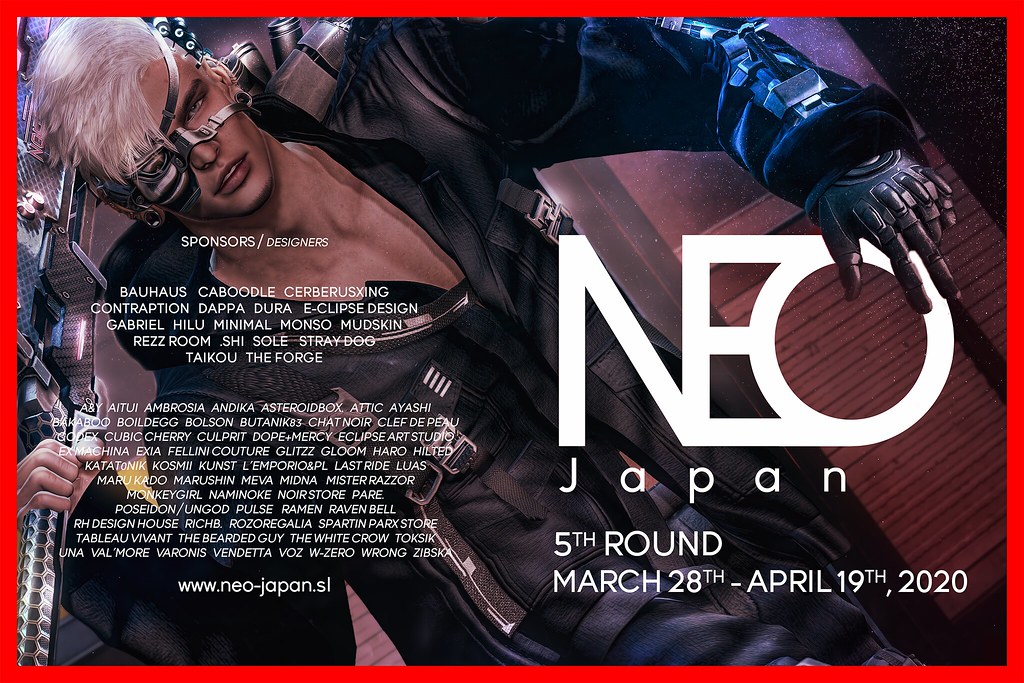This detailed photograph features a striking magazine cover promoting "NEO Japan 5th Round," dated March 28th to April 19th, 2020, with the URL www.neojapan.sl. Dominating the left side of the image is a character with short, white platinum hair and a distinctive steel eye patch covering her left eye and partially her cheek. This eye patch extends over her nose and around to her right ear, with an additional metal piece encircling her head. She is dressed in a black jacket with a V-neck, partially covering a bionic silver arm on her right side. Held in her other hand is a large sword with a silver and black embroidered handle, accentuated by pink lights. The character is also seen with black pants and various weapons or tools near her left torso. Other key elements include the red outline of the poster and a section listing sponsored designers. Text on the cover mentions the event details and sponsors but is partially obscured by the character's positioning.